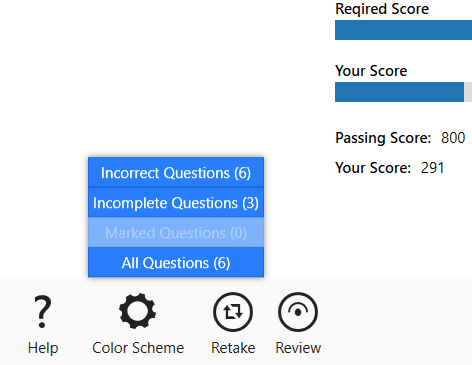This image appears to be a detailed screenshot of a scoring system interface. In the upper right-hand corner, a horizontal progress bar is displayed, accompanied by text labels. The first label, "Required Score," is in black text above a completely filled navy blue bar. Below it, another label, "Your Score," is also in black text, with its corresponding bar approximately 95% filled in navy blue, leaving a small segment in light gray. The text indicates the "Passing Score: 800," while "Your Score" is at 291.

In the lower left-hand corner, there is a section listing different categories of questions. Each category is on a blue row with white text: "Incorrect Questions (6)," "Incomplete Questions (3)," "Marked Questions (0)," and "All Questions (6)."

At the bottom of the screenshot, on a light gray background, several icons and options are available. From left to right, there is a question mark icon with "Help" written beneath it, a gear icon labeled "Color Scheme," a circular icon featuring an upward and downward turning right angle with arrows and labeled "Retake," and finally, an eyeball icon with an eyelash labeled "Review."